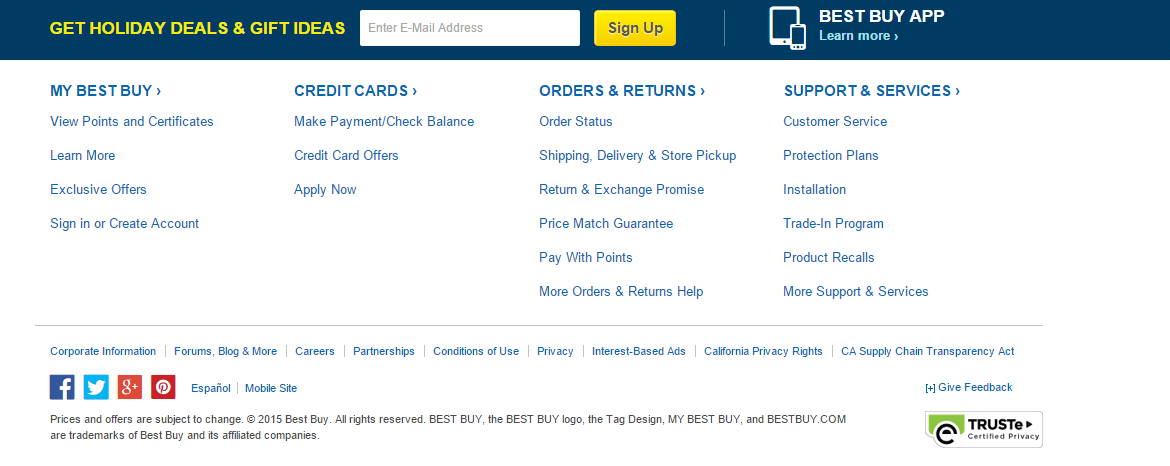The image is a promotional banner from Best Buy's website that highlights various features and services available to customers. 

At the top, there is a prompt in gray text within a data field that says "Enter email address." To the right of this field, a vibrant yellow button displays the text "Sign Up." Adjacent to the email sign-up area, the phrase "Best Buy app, learn more," is present, along with the message "You're at Best Buy."

Beneath this section, a strip of dark green-blue or teal color showcases the text "Get holiday deals and gift ideas" in yellow. Further down, set against a white background with teal-colored font, the following sections are outlined:

- **My Best Buy**: Options to view points and certificates, access exclusive offers, and sign in or create an account.
- **Credit Cards**: Information on making a payment, checking balance, credit card offers, and applying now.
- **Orders and Returns**: Details about order status, shipping and delivery, store pickup, return and exchange promise, price match guarantee, paying with points, and additional help for orders and returns.
- **Support and Service**: Customer service, protection plans, installation services, trade-in programs, product recalls, and additional support and services.

Separating these sections and the bottom navigation is a gray line. The navigation line includes corporate information starting on the left, covering topics such as corporate information, forums, blogs, careers, partnerships, terms and conditions of use, privacy policies, interest-based ads, California privacy rights, and the California Supply Chain Transparency Act.